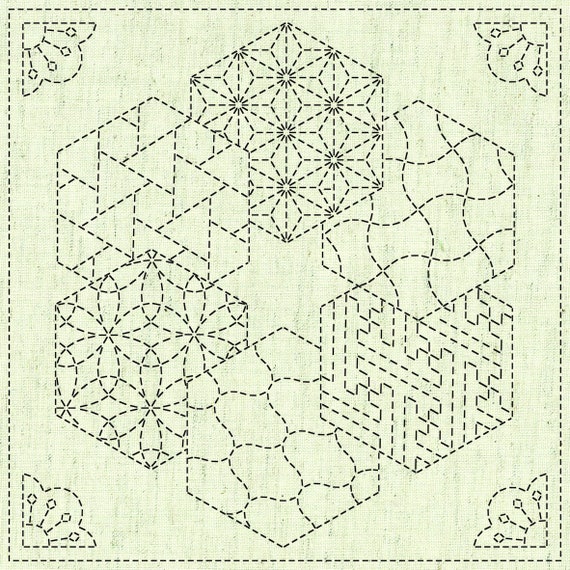This detailed illustration presents a complex geometric design rendered in black dotted lines against a rough white background peppered with black spots. At its core, the design features six hexagonal shapes arranged to form a larger hexagon, each adorned with unique interior patterns of wavy and floral lines. Surrounding this central hexagonal motif is a square border, also created with dotted lines, suggestive of stitching or sewing guides, which hints at this being a conceptual pattern for a sewing project, like a quilt or blanket. At each of the four corners of the square border, there are fan-shaped decorations, featuring circular and linear motifs, further unified by the dotted stitching theme. The entire image maintains a consistent light gray color scheme, enhancing its intricate details and the cohesive use of dotted lines throughout.